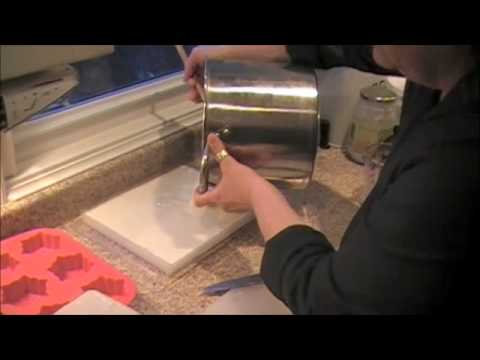In the image, a Caucasian woman, possibly elderly, is seen in a kitchen near a window and sink, indicated by a visible tea kettle in the background. She is wearing a black long-sleeve shirt and a gold ring on her left thumb. Her pale arms and a portion of her chin are visible as she holds a large, silver-colored metal pot with both hands, pouring a liquid onto a white tray positioned on a brown granite countertop. To the left of this scene is a distinctive red-pink mold with hexagonal or leaf-shaped compartments, presumably for baking or candy-making. The kitchen scene is slightly blurry but rich in detail.